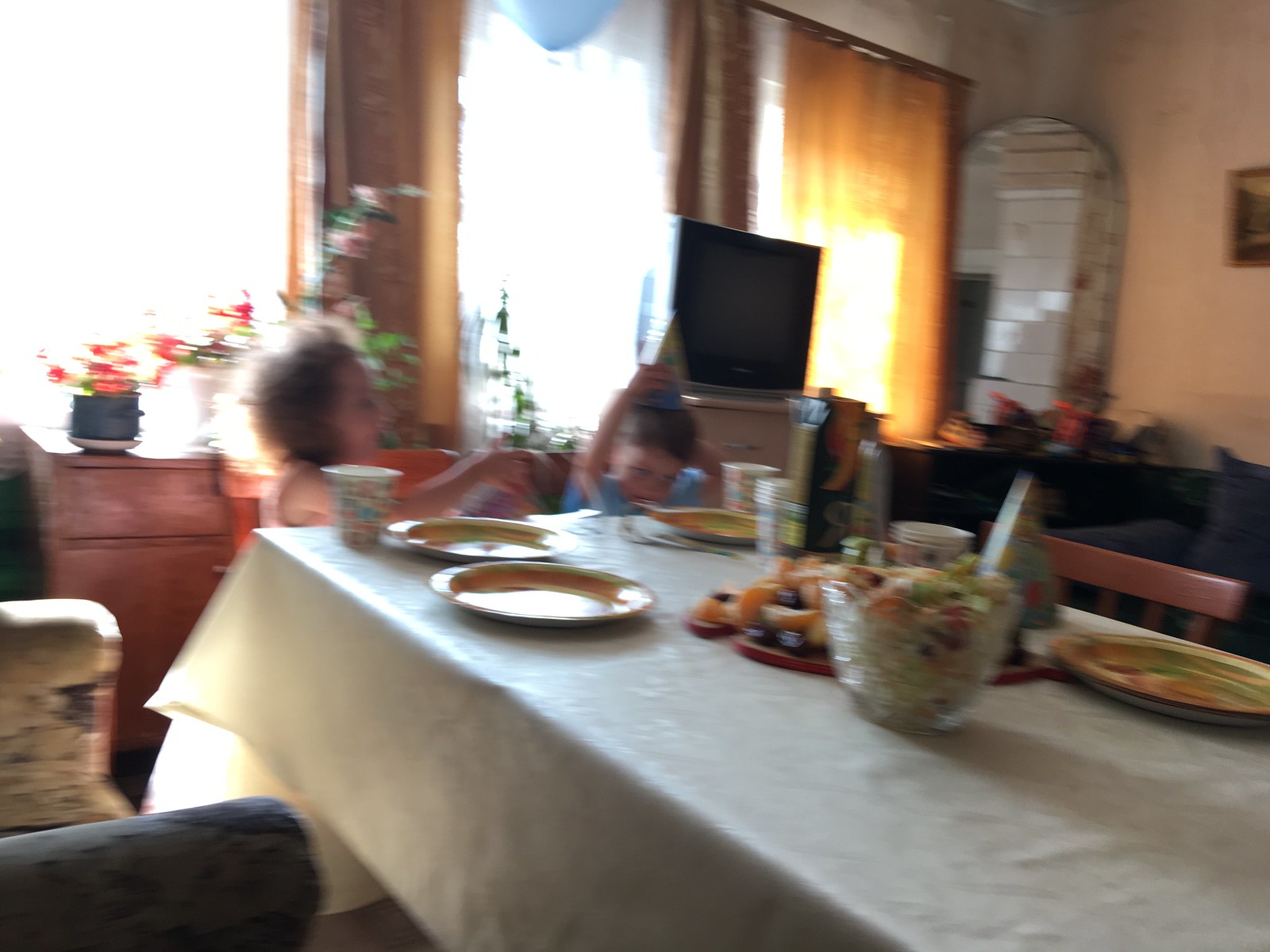In this blurry photograph, a cozy, older home interior is depicted. The table, covered with a white tablecloth, holds a plate of fruit, several paper plates, and a paper cup, hinting at a festive gathering. Bright light filters through the curtained windows, illuminating the scene. An old television, not a modern flat screen, sits in the background, adding a touch of nostalgia. Visible through a curved archway is another room with a blue sofa and a blue chair on the left.

The main focus of the photo is on two out-of-focus figures in motion: an older woman with curly brown hair and a child dressed in a blue shirt, possibly a boy, though their rapid movement blurs their features. The child appears to be putting on a cone-shaped birthday hat, suggesting this is a celebratory moment. The blur of movement and the presence of party items like paper plates and a cup contribute to the lively, yet nostalgic atmosphere of this image.